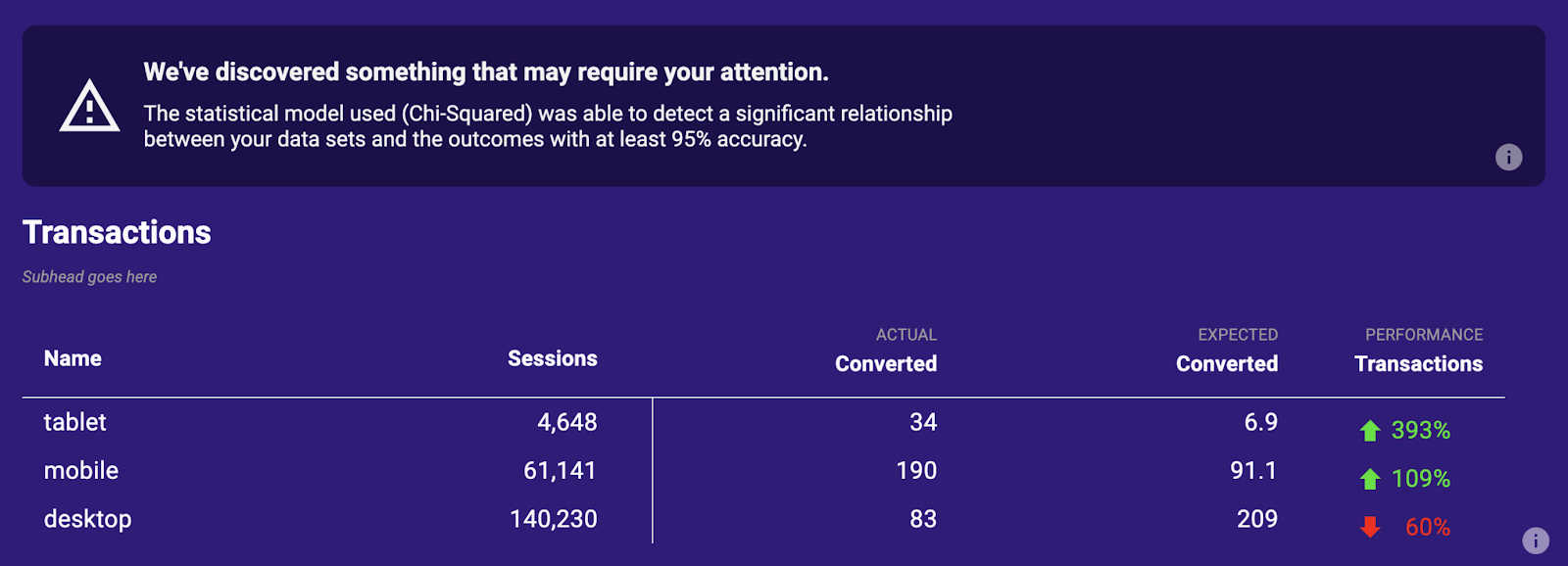The image showcases a screenshot with a deep purple background. At the top, there is a black rectangle containing a message. Inside the black rectangle, a white-outlined black triangle with a white exclamation point symbol is prominently displayed. The message reads: "We've discovered something that may require your attention. The statistical model used (χ²) was able to detect a significant relationship between your data sets and the outcomes with at least 95% accuracy." 

Below the message, there is a gray circle with a lowercase "i" inside, indicating additional information. As you scroll down, the section headers "Transactions" and "Name" are clearly visible, followed by columns labeled "Sessions," "Converted," "Actual Converted," "Expected Converted," and "Performance Transactions." On the right side of the screen, green up arrows with corresponding percentages and a red down arrow with a percentage are displayed, indicating the performance metrics.